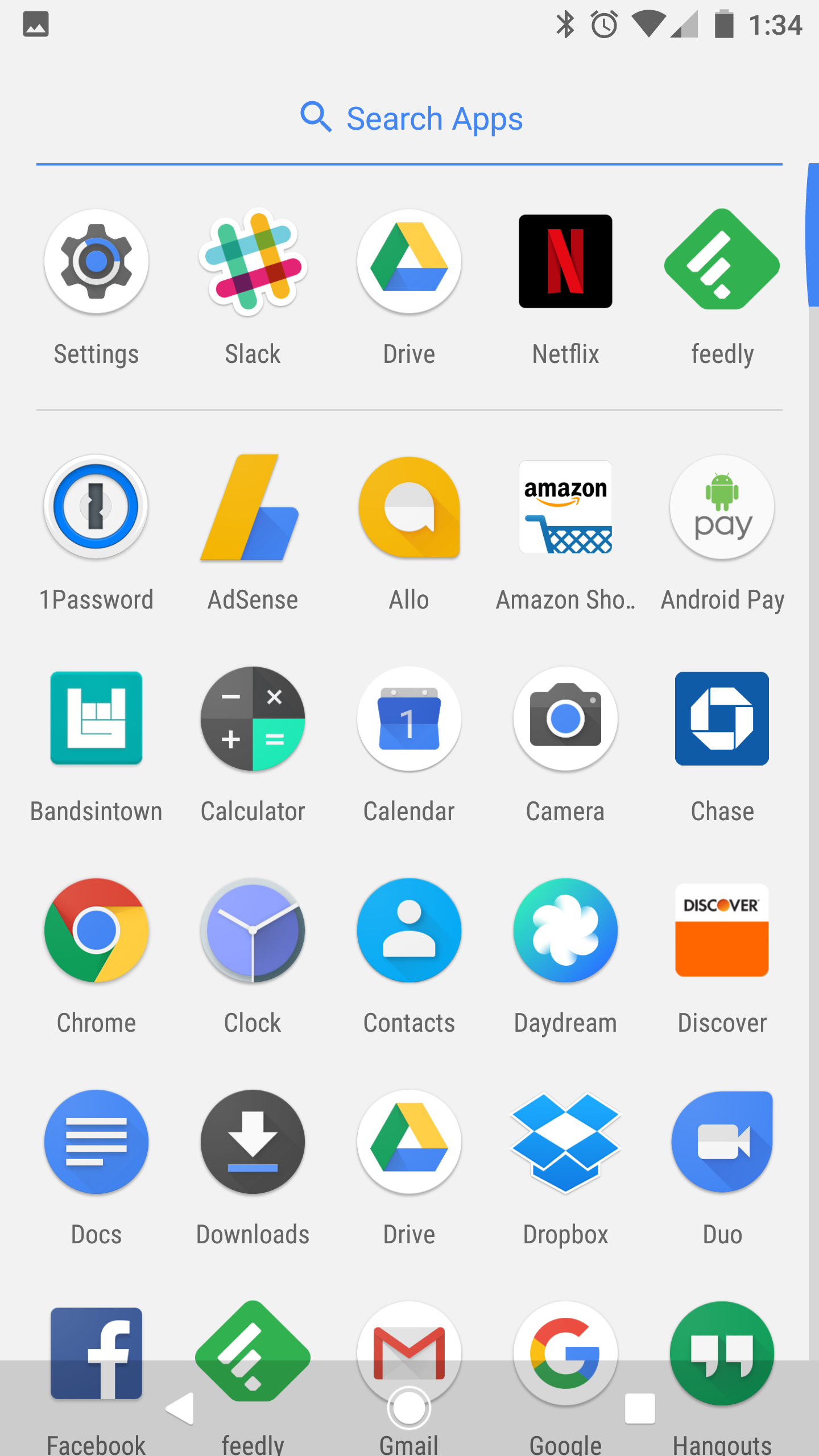This is a detailed screenshot of a mobile app page captured on a phone with a white background. The rectangular screenshot displays various phone interface elements along the top edge. On the left side, there's a dark gray icon for Bluetooth, followed by a phone icon, and then a series of Wi-Fi bars that are fully filled in dark gray, indicating strong connectivity. The phone signal bars, in contrast, show a low signal strength with minimal filled sections. Adjacent to these is the battery bar, which is almost full, represented by a dark gray color. To the far right, the current time is displayed as 1:34.

In the upper central part of the image is the "Search apps" option, consisting of a magnifying glass icon next to the text "Search apps" in blue. This section is separated from the rest of the image by a long horizontal line.

Below this line, a comprehensive list of the person’s apps is visible, each labeled in medium gray text with corresponding circular icons. Some of the apps include Settings, Slack, Drive, Netflix, Feedly, 1Password, AdSense, Allo, Amazon Shopping, Android Pay, Bandsintown, Calculator, Calendar, Camera, Chase, Chrome, Clock, Contacts, Dream, Discover, Docs, Downloads, Dropbox, Duo, Facebook, Gmail, Google, and Hangouts. The layout clearly organizes the apps, making it easy to identify each by both name and icon.